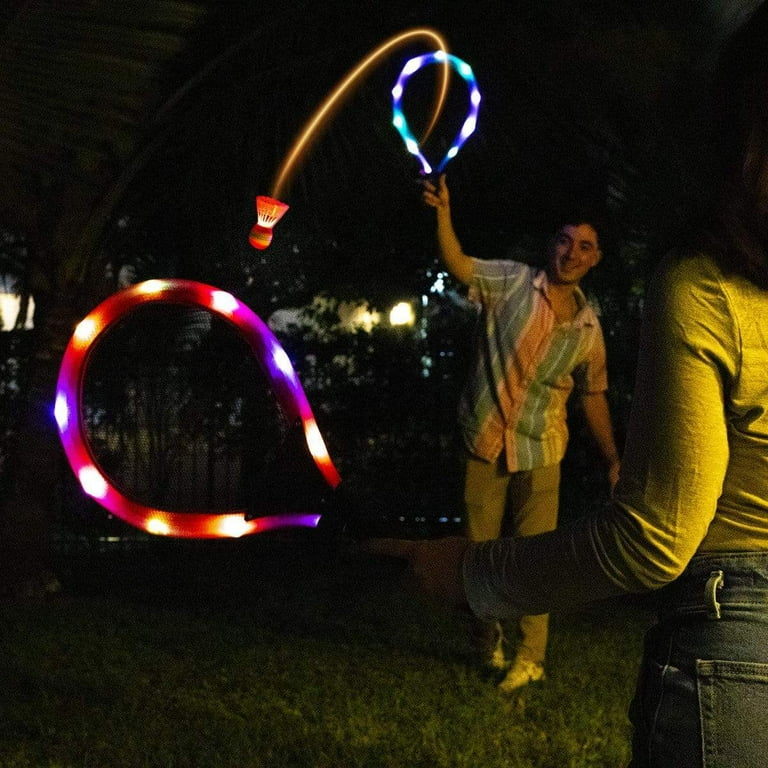In an image taken in the dark, two individuals, a white male and a female, are engaged in a game of badminton using illuminated equipment. The man, wearing cargo pants, sneakers, and a pink and blue striped collared shirt, is in the active motion of hitting a brightly lit red shuttlecock towards the woman, who is dressed in jeans and a long-sleeved shirt and is facing away from the camera. They each wield neon-lit rackets, one blue and one pink, that have lights outlining the edges. The vibrant lights of the rackets and shuttlecock dominate the scene, casting colorful glows in an otherwise dimly lit, fenced backyard, possibly at night. The backdrop is faint but includes a visible palm leaf in the top left corner, adding more context to the outdoor setting. The pair appears to be having fun, possibly at a party, enjoying their luminous playthings in the darkness.